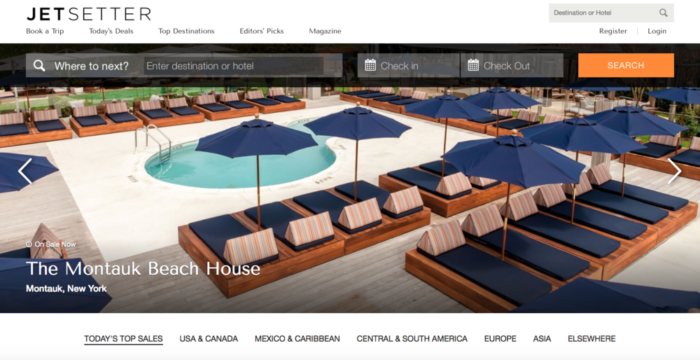In this screenshot set against a solid white background, the upper left corner features the website name "Jet Setter" with the word "Jet" bolded. Navigational options such as "Book a Trip," "Today's Deals," "Top Destinations," "Editor's Picks," and "Magazine" are listed prominently. The upper right corner includes a search bar with options to register or log in. Below this, a black banner offers a "Where to Next?" search function, prompting users to enter their desired destination or hotel. This search area includes fields for check-in and check-out dates, each with an accompanying calendar icon, and an orange "Search" button for action.

The central focus of the screenshot is a vibrant photo of Montauk Beach House in Montauk, New York, with the text "On Sale Now" displayed in small white letters above the image. The photo captures a stunning scene featuring a kidney-shaped swimming pool surrounded by elegant lounge chairs. These chairs rest on what appears to be cedar wood platforms, each adorned with blue cushions and striped pillows in shades of orange, gray, and beige. Scattered between the chairs are large blue umbrellas, each mounted on wooden poles that match the platforms, creating a harmonious and inviting atmosphere.